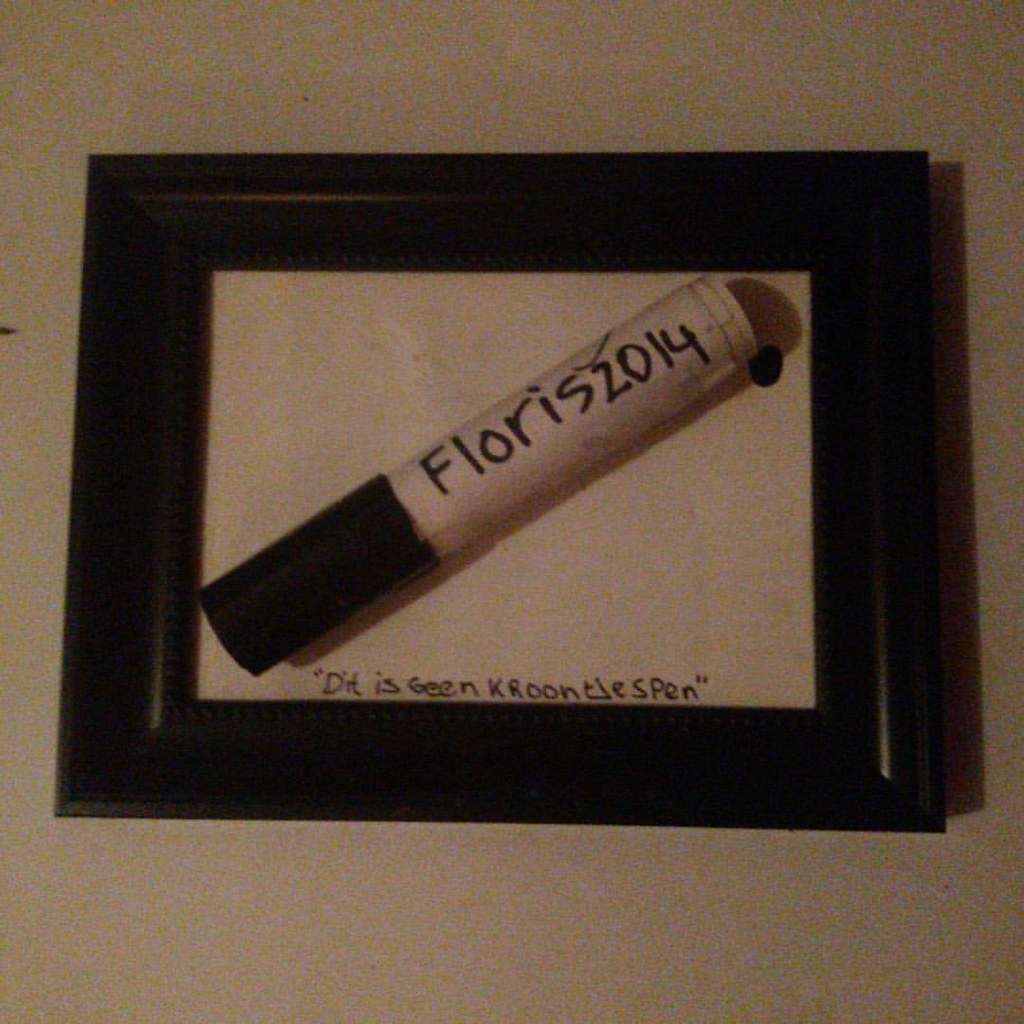This image showcases a rectangular black picture frame, likely made of wood, displayed on a stark white surface. Centrally positioned within the frame is what appears to be a white marker, capped with black. The marker is inscribed with "FLORIS2014" in prominent lettering. Below this, a less comprehensible text reads "DIT IS GEEN KROONSJESPEN," with the phrase enclosed in quotation marks. The overall composition presents a contrast between the black frame and the white surface, with the marker artfully angled inside, making it ambiguous whether the art is a flat picture or a three-dimensional object.